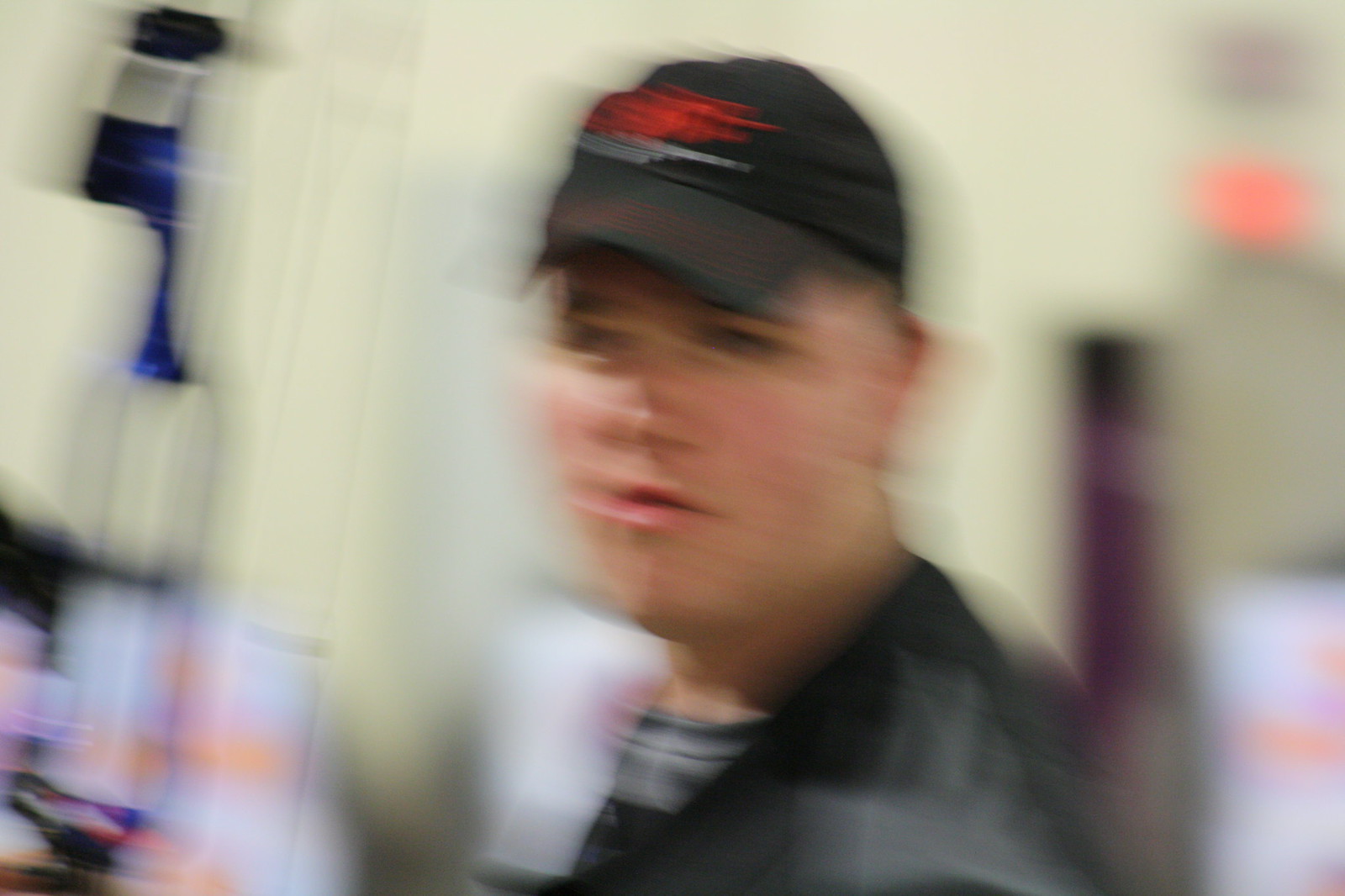This highly blurred photograph features a young man captured in a side profile. He stands with his chest angled towards the left side of the image and his face turned partially towards the camera. He dons a black hat with red writing adorning the top, and a white towel is draped over his left shoulder. The man is dressed in a black vest over a black and gray t-shirt. Although the image lacks focus, a glowing exit sign is visible in the top right corner. Additionally, to the left of the man, there appears to be a drink machine, characterized by what seems like a stack of cups. The man’s youthful face, squinty eyes, and slightly open mouth are faintly discernible despite the poor quality of the image.